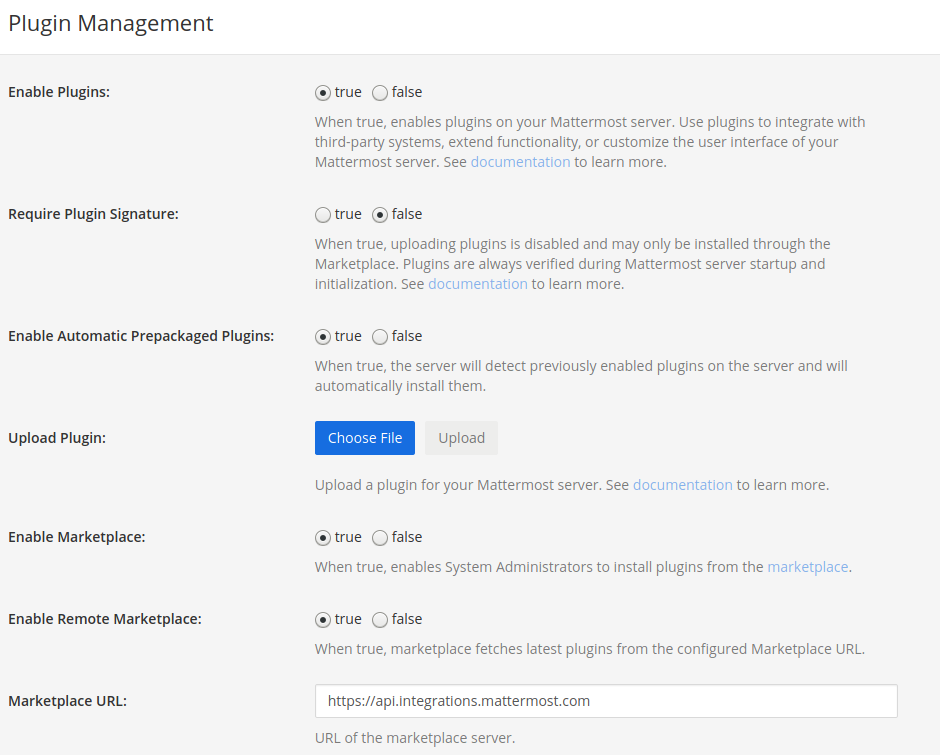### Detailed Caption for Plugin Management Settings Image

The image illustrates the "Plugin Management" settings interface for a Mattermost server, highlighted by a black heading at the top. Below this heading, there's a light gray rectangular section containing a grid of columns, each with specific plugin-related configurations.

From left to right, the columns under the black header are as follows:

1. **"Enable Plugins"** - This column has a check box marked as "true." When set to true, it enables plugins on your Mattermost server, allowing integration with third-party systems, extension of functionality, or customization of the user interface. A blue hyperlink labeled "documentation" is provided for further details.
   
2. **"Require Plugin Signature"** - The option in this column is marked as "false." When true, it restricts plugin uploads, making them installable solely via the marketplace. Plugins undergo verification during Mattermost server startup and use, with further details available through a blue "documentation" link.
   
3. **"Enable Automatic Prepackaged Plugins"** - This check box is also marked "true." When activated, the server detects any previously enabled plugins and installs them automatically.
   
4. **"Upload Plugin"** - This section features a blue button labeled "Choose File" and a gray "Upload" button, accompanied by a note to upload a plugin for your Mattermost server, directing users to a blue "documentation" link for more information.
   
5. **"Enable Marketplace"** - The check box here is marked "true." When enabled, system administrators can install plugins from the "Marketplace," which is highlighted in blue.
   
6. **"Enable Remote Marketplace"** - This option is also marked "true." When enabled, it allows the marketplace to fetch the latest plugins from the configured marketplace URL.
   
7. **"Marketplace URL"** - This column specifies the URL for the marketplace server, ensuring the most recent plugins are available for installation.

Each setting provides an option to toggle between true or false, facilitating customized plugin management for the server administrators.